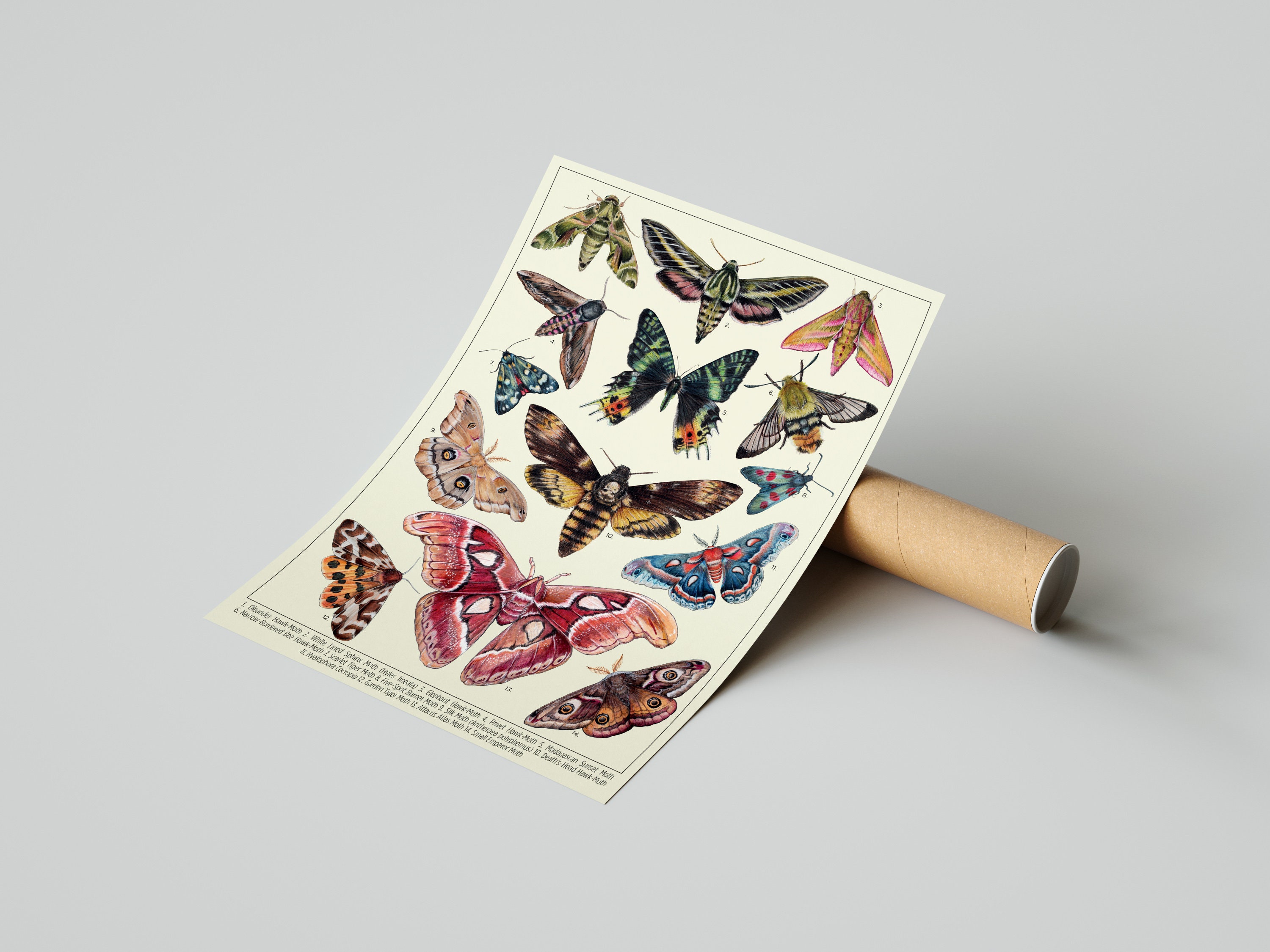This image features a vertical, 11-inch by 17-inch botanical poster displaying 14 vibrant, multicolored moths and butterflies. Each insect is uniquely adorned with intricate wing patterns, showcasing a spectrum of colors including emerald green, rosy pink, oranges, reds, blues, and browns. These detailed illustrations resemble traditional botanical drawings, exuding an antique charm. The background of the poster is an ivory hue, framed by a black outline. At the bottom, there are three lines of small text likely describing the various species depicted. The poster is propped against a brown, round symmetrical tube, all set on a pristine, white surface. The photograph capturing this scene is taken from an above angle, approximately 65 degrees, providing a comprehensive view of this stunning and detailed display.